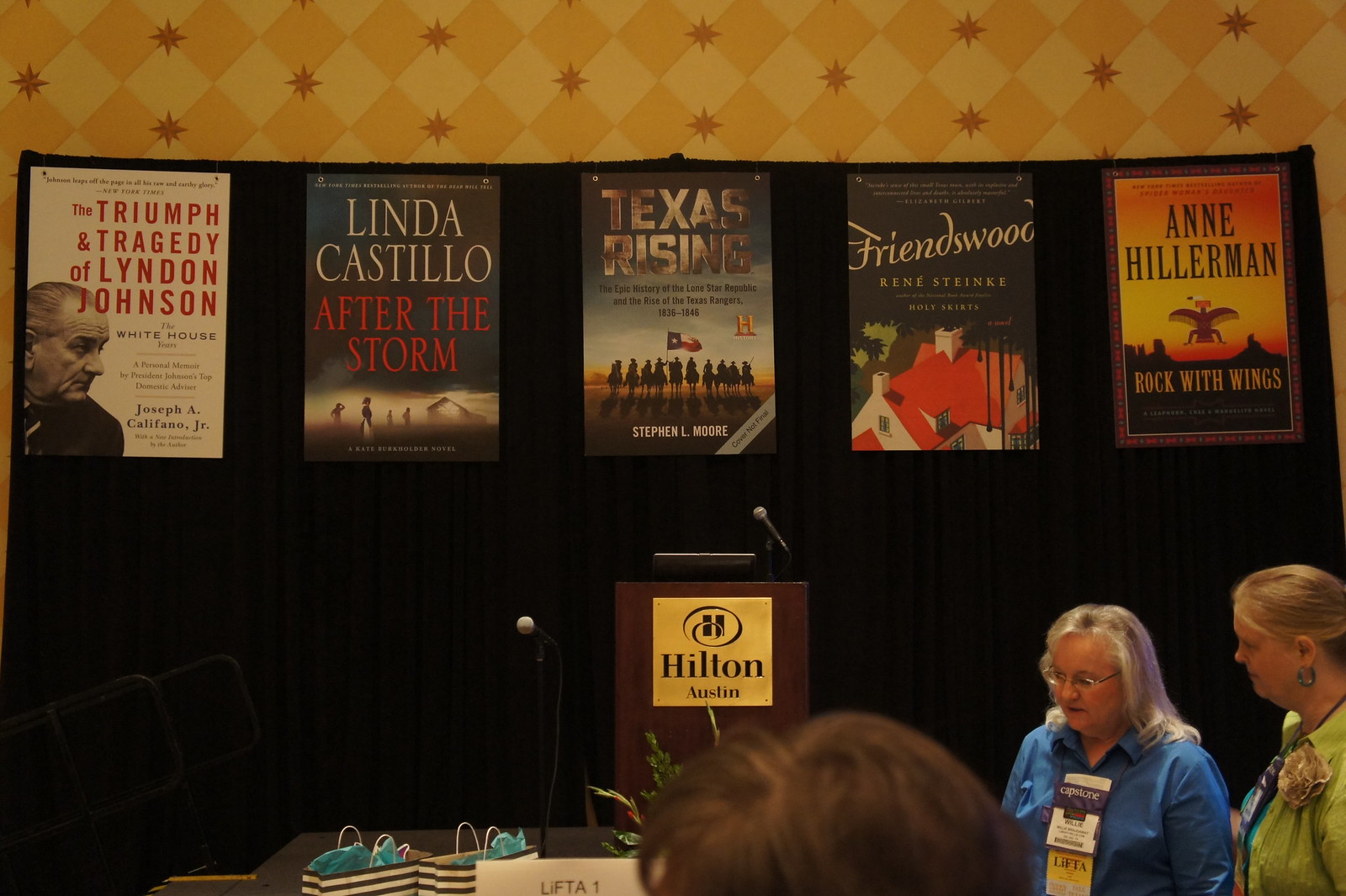This photograph, likely taken at a literary or publishing conference, features a wooden podium centrally positioned with a golden plaque reading "Hilton Austin" and equipped with a microphone, but currently unattended. Directly in front of the podium, red flowers are placed, and to the left are black and white striped gift bags adorned with blue tissue paper. Above the podium, five posters display the covers of various books: "The Triumph and Tragedy of Lyndon Johnson," "After the Storm" by Linda Castillo, "Texas Rising," "Friendswood," and "Rock with Wings" by Anne Hillerman. In the foreground, partially visible at the bottom of the image, is the back of an attendee's head. Further to the right, two elderly women are walking across the scene; one has white hair and is wearing a blue blouse with a placard, while the other has blonde hair and is dressed in a green blouse. The indoor setting features a black backdrop, with a color palette that includes yellow, red, gray, gold, blue, and green.